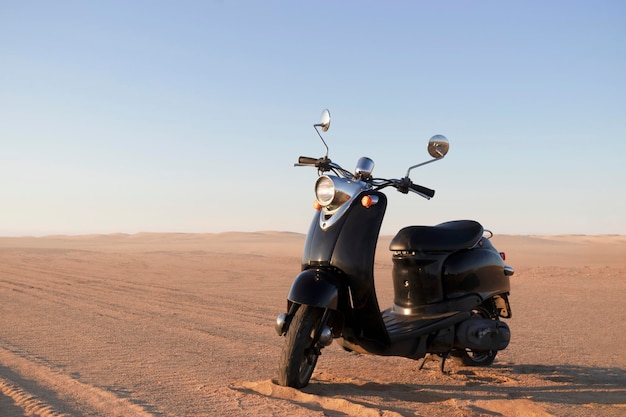The photograph captures a sleek, black motor scooter prominently positioned in the bottom right corner of a sunlit desert landscape. The foreground reveals tire tracks in the lower left corner, hinting at movement across the sandy, featureless expanse. The scooter stands upright on its kickstand, its polished black metal body glinting in the abundant daylight. The front boasts a chrome headlight casing, flanked by two yellow turn signal lights, and a pair of round metal rearview mirrors extending from the handlebars. A long, padded seat extends back to the small black fender, embodying a modern aesthetic that suggests it was manufactured within the last two decades. The surrounding desert stretches to a low, rolling horizon at the halfway mark of the frame, under a bright, yet subtly faded blue sky. The absence of people, identifiable markings, and a clear, high-quality image indicate that this could be a computer-generated depiction, meticulously detailed to evoke a real-life scene.